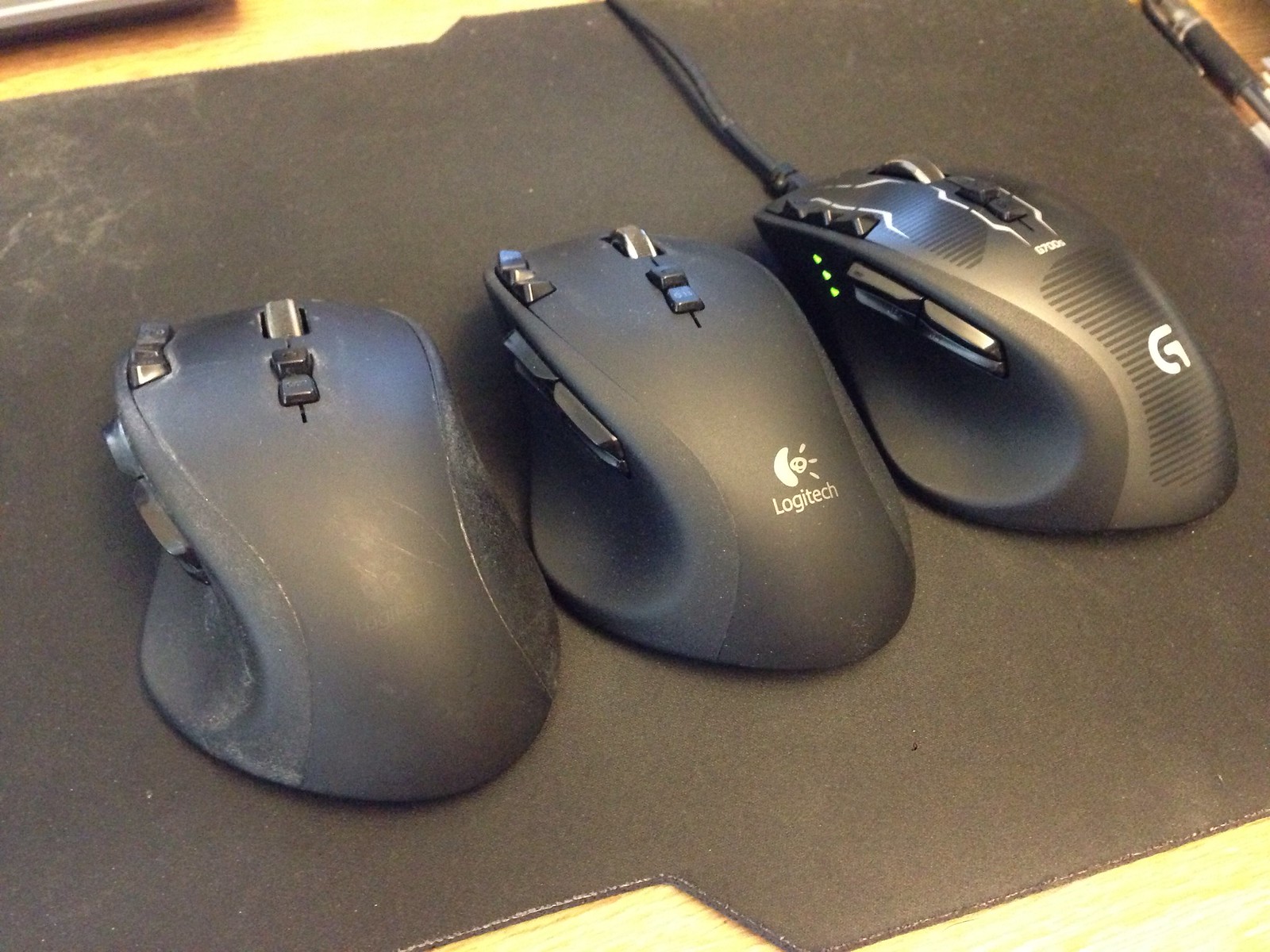The image depicts a color photograph of three computer mice aligned side by side on a black mouse mat with irregular cutouts, revealing a wooden desk underneath. Starting from the left and moving diagonally to the right-hand corner of the frame, the first two mice are wireless, while the third is wired, with the cord extending forward away from the viewer. The mouse in the center bears the white text "Logitech" and a silver logo above it. The rightmost mouse, featuring a distinct white letter "G" on its back, has additional silver patches and three green LEDs on the left side, indicating battery status. All three mice are primarily black and equipped with multiple buttons, including side, thumb, and scroll buttons. The setup sits under indoor lighting, with a partially visible pen in the upper right corner of the frame. The mice and the mouse mat show signs of wear and dust, suggesting frequent use. The detailed design and additional buttons of the mice hint at their suitability for advanced or gaming purposes.